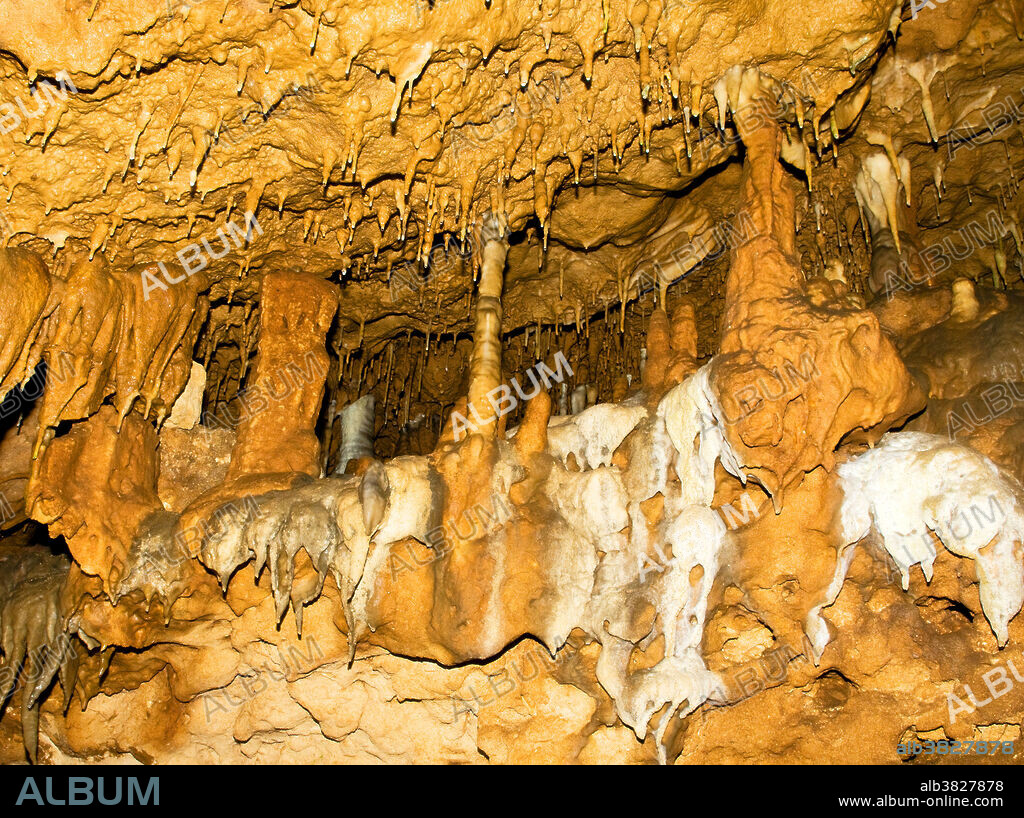Inside a cave, this image captures an intriguing scene of mineral formations that appear to drip from the roof. The cave's ceiling, which occupies the top fourth of the image, is adorned with stalactites—elongated, icicle-like structures that give the impression of a muddy, wet texture that once oozed and then solidified. These formations, primarily in hues of tan, dark brown, and white, create a fascinating contrast against the rocky backdrop. Toward the top, some pillar formations lead back into a smaller cavern or pocket, with white stalactites dripping down from above. In the bottom third of the image, the cave floor is visible, completing the scene's composition with a rugged texture. 

Adding to the mystique, text overlays the image: the word "ALBUM" is prominently displayed in gray on a black border at the bottom, along with a sequence of letters and numbers, "ALB 3827 878." Additionally, the text "www.album-online.com" appears meticulously printed in small white letters, enhancing the photo's unique presentation. This detailed description encapsulates the raw beauty and distinctive features captured within the cave's subterranean environment.